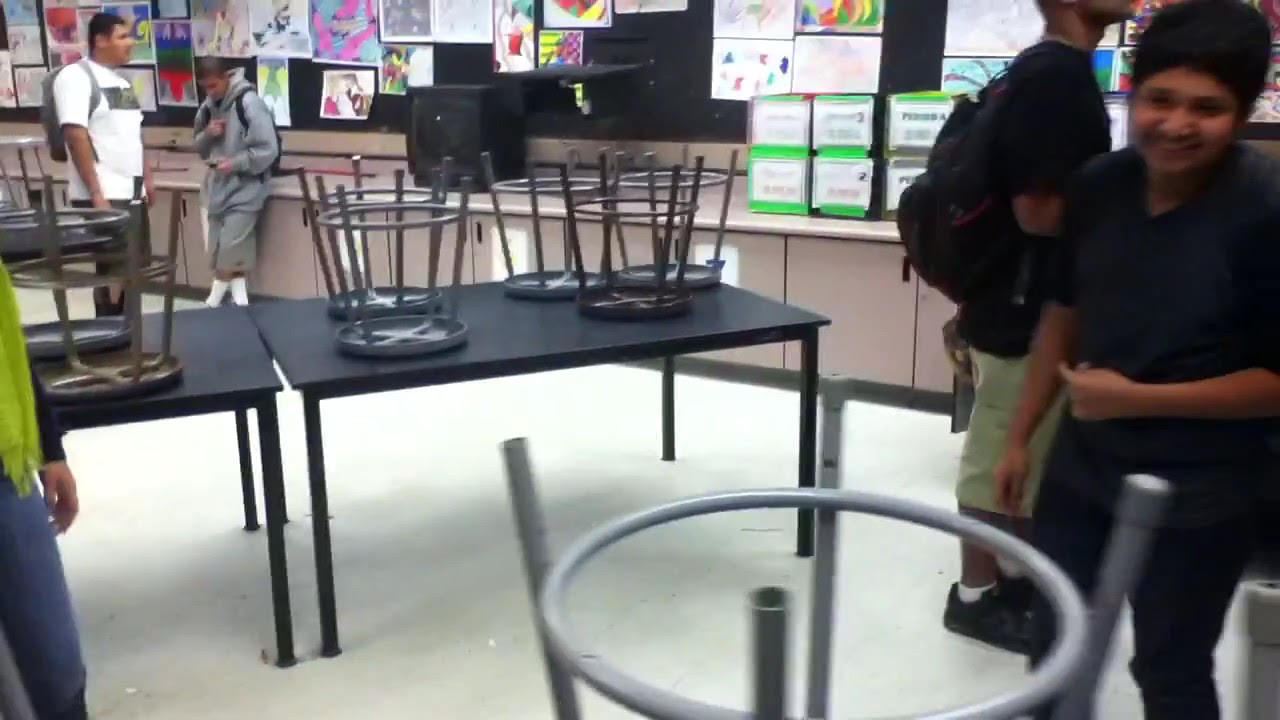In the image, a little boy stands in what appears to be an art classroom. He is wearing dark pants and a dark shirt, with another boy behind him dressed in a dark shirt, green shorts, and carrying a dark backpack. The room is filled with other children and features several dark-colored tables with upside-down stools on top. The floor is light-colored, and the walls are adorned with multicolored drawings, likely created by the students. There's an old TV visible on one of the tables. The setting is bustling with activity, as multiple students can be seen laughing and talking among themselves. The arrangement of objects and people indicates that the classroom is designed for creative activities, providing a vibrant and dynamic environment for the kids. The scene is likely captured during a school day, with the majority of the action taking place to the right and left sides of the room, and the tables centrally positioned.